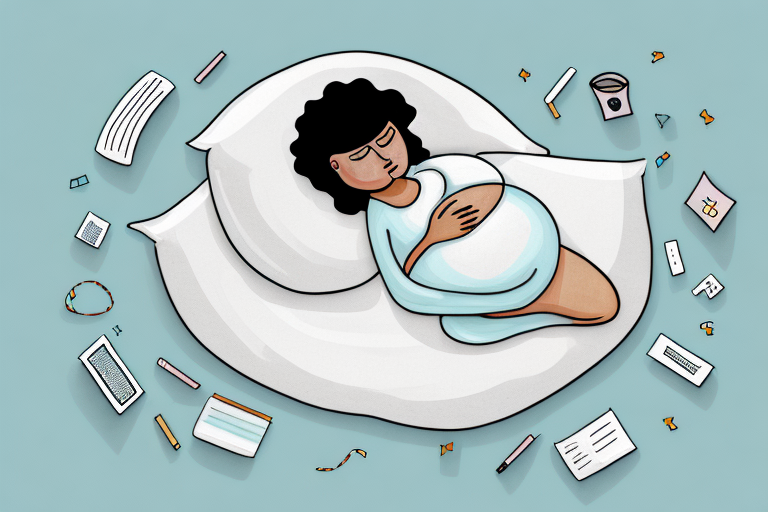This image features a detailed drawing of a very pregnant woman lying on a large, fluffy bed or body pillow. The pillow, which looks incredibly soft and comfortable, supports her head with an additional smaller pillow. The woman, dressed in a blue nightgown, has her hands gently resting on her prominent belly. Her black hair, illustrated with wavy, curly lines, frames her abstractly drawn face, which sports simple rectangular eyes. One of her legs appears to be tucked underneath her, adding to her relaxed, reclined posture.

Surrounding her, from around 11 o'clock to 1 o'clock if visualized as a clock face, are various scattered items that enhance the scene's layered complexity. These include a mix of what seems to be medical supplies, a bracelet, prescription forms, and even broken cigarettes. There are also numerous small pieces of paper, resembling confetti or stationery supplies, spread around. The entire setting is displayed against a light blue background, accented by the main colors of black, peach, and white, contributing to the artwork's cohesive and tranquil aesthetic.